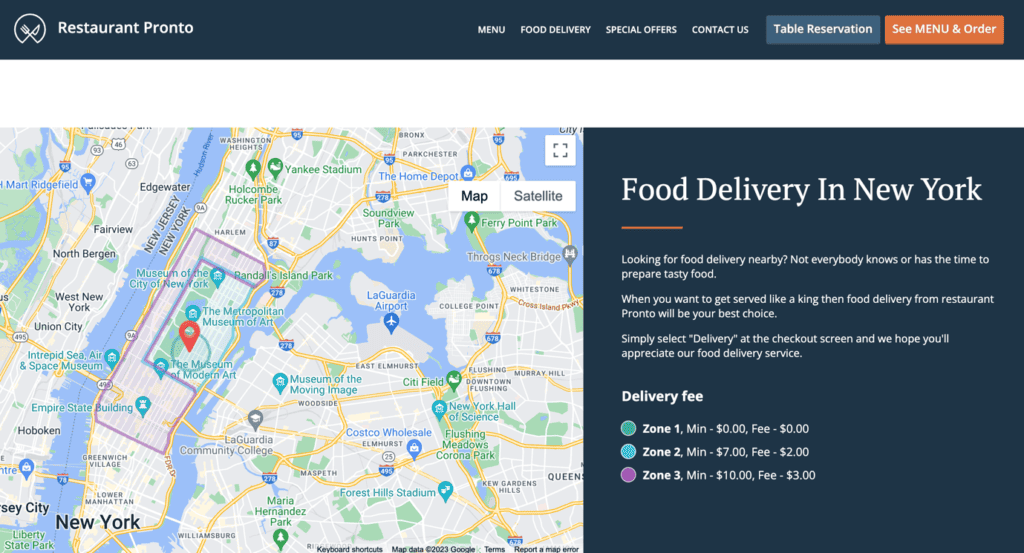The top section of the image features a black navigation bar with a partially visible circle on the left side, containing a small stylized icon resembling a fork and either a knife or spoon. Next to this icon, the restaurant’s name "Restaurant Pronto" is displayed in white text. To the right of the name, white text links labeled "Menu," "Food Delivery," "Special Offers," and "Contact Us" are aligned horizontally. Below the navigation bar, a dark gray box with white text reads "Table Reservation." Adjacent to this, an orange box with white text prompts viewers to "See Menu and Order."

Beneath these elements, there is a Google Maps screenshot of New York City, highlighting the central area of Manhattan with a red push pin that marks Restaurant Pronto’s location. 

On the right side of the image, a black box with a white header reads "Food Delivery in New York," accented by a small orange line beneath the header. Below this, white text states: "Looking for Food Delivery Nearby? Not everybody knows or has the time to prepare tasty food. When you want to get served like a king, then Food Delivery from Restaurant Pronto will be your best choice."